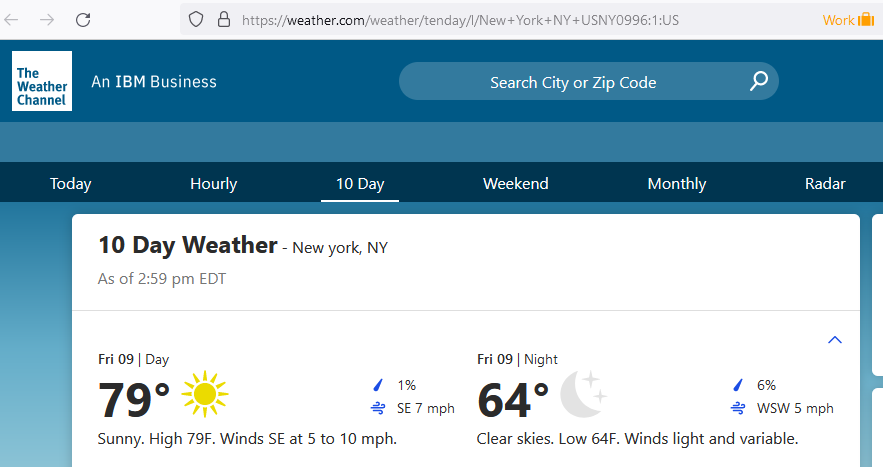This image showcases a detailed view of a weather webpage. At the very top is the browser’s address bar, featuring the left and right navigation arrows, a reload button, and an address field that displays a shield icon and a padlock icon, indicating a secure connection. The URL in the address bar reads: "https://weather.com/weather/tenday/i/new+york+ny+usny0996:1:us." To the right of the address bar is a yellow label with the word "Work" accompanied by a suitcase icon.

Below the address bar, the webpage displays a header with a blue background. On the top left is The Weather Channel logo, with the tagline "An IBM Business" positioned next to it. Centrally located on the header is a search bar with the placeholder text "Search City or ZIP Code" and a magnifying glass icon.

The webpage header is followed by navigation tabs on a darker blue banner: "Today," "Hourly," "10 Day," "Weekend," "Monthly," and "Radar," with the "10 Day" tab being highlighted and underlined, indicating the current selection.

Beneath this banner, bold text announces "10 Day Weather - New York, NY" followed by the updated time "As of 2:59 PM EDT." This section features a white background. Below these details, there is a segmented forecast for Friday, aligned horizontally. Starting with the daytime forecast, it displays:

- "Friday 09, Day: 79°F" with a sun icon indicating sunny conditions.
- The description reads: "Sunny. High 79°F. Winds SE at 5-10 mph."

Next is the nighttime forecast for Friday:

- "Friday 09, Night: 64°F" with a moon icon indicating clear skies.
- The description includes: "6% chance of rain. Winds WSW at 5 mph, clear skies. Low 64°F, winds light and variable."

Overall, the image provides a comprehensive view of a weather forecast webpage, showcasing various elements from browser features to detailed weather predictions for New York, NY.